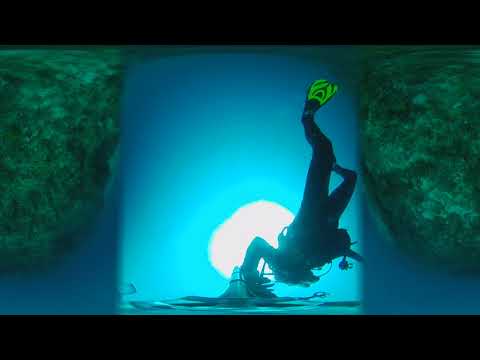The image is a horizontally aligned rectangular underwater color photograph featuring a diver dressed in all-black scuba gear with bright neon green flippers. The diver is in an upside-down position, appearing to dive downwards with their legs up. The image quality is somewhat blurry, making finer details hard to discern. Central to the composition is a large, bright circle, which could be an entrance or exit to a tunnel, emanating light amidst the generally blue-hued water. On both the left and right sides of the image, there are large, roundish grey-green rocks or possibly underwater vegetation, partially framing the diver in the middle. These surrounding elements create a darker blue shade around the diver, who seems to be touching or grabbing something on the ocean floor. The photograph is bordered by thick black bars at the top and bottom, suggesting it might be a still captured from a video. The perspective is slightly disorienting, giving an impression of a flattened 360-degree view with the bright light in the middle resembling the Sun as seen from underwater.